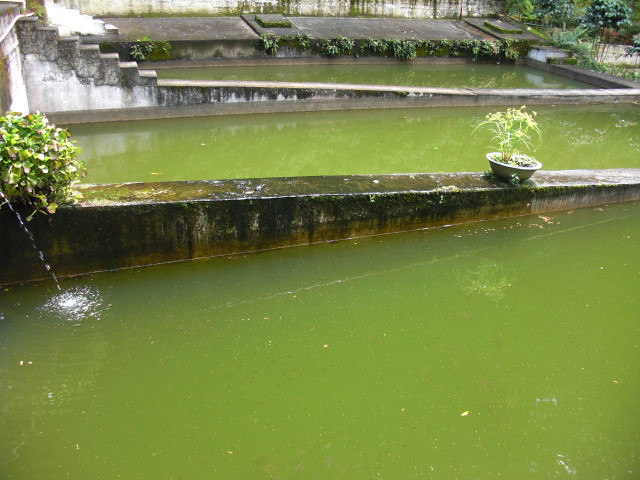The photograph showcases a segmented, man-made pond with distinctly green water, separated by aged, mossy concrete barriers. The barriers are stained, sloping, and detailed with patches of black mold, indicating their age. Towards the back of the image, one barrier features narrow stair steps, while others host small potted plants. In the upper left corner, a small stream of water is seen shooting out from an unseen source, causing splashes in the pond. The background reveals a white, moss-covered wall with additional shrubbery at the very top, adding to the scene's lushness. The layout suggests a wide, vertical, rectangular composition, with the concrete structures narrowing from left to right, creating a layered, pathway-like appearance. The overall setting appears serene and devoid of people, hinting at the possibility of it being a private property rather than a public park.